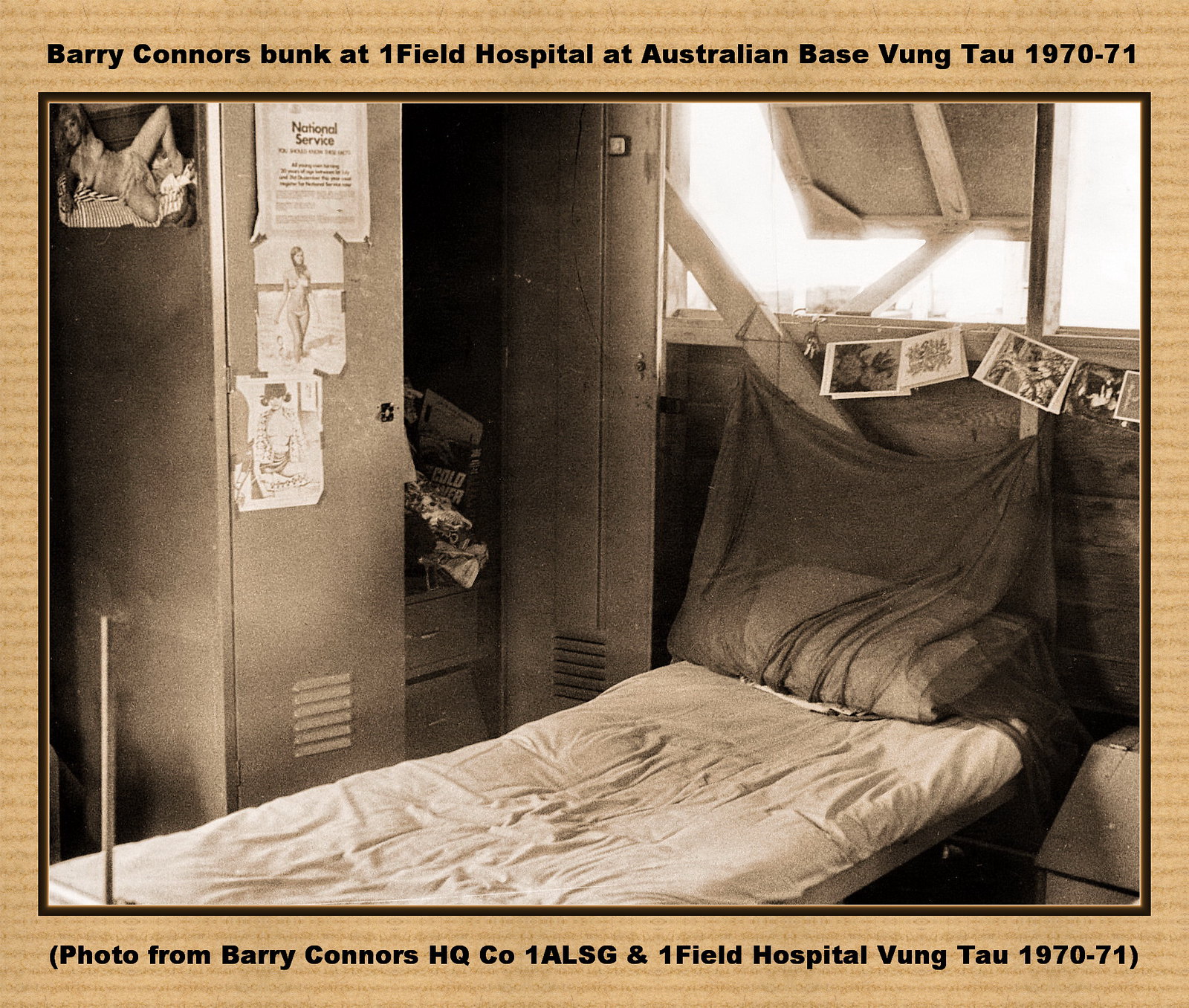This sepia-toned photograph shows a modest military bunk room at the Onefield Hospital, located at an Australian base in Vung Tau, during the years 1970-71. Central to the image is an unmade long cot with a thin mattress, covered by a white blanket and a pillow overlaid with a black net, probably serving as a mosquito net. The bed is positioned beneath a partly open window, held ajar by a small wooden beam. Above the cot hang a series of postcards and cards, likely sent by loved ones. To the right of the cot, an open locker reveals an assortment of blankets and books. Scattered on the locker are pieces of paper and photographs, including what appear to be pin-up images. The wooden structure of the cabin suggests a rustic, utilitarian design. The photograph is framed in a beige border with dark horizontal striping, adorned with two captions in bolded sans-serif font. The top reads "Barry Connors’ Bunk at Onefield Hospital at Australian Base, Vung Tau, 1970-71," while the bottom states "Photo from Barry Connors Headquarters, CO, 1ALSG and Onefield Hospital, Vung Tau, 1970-71."